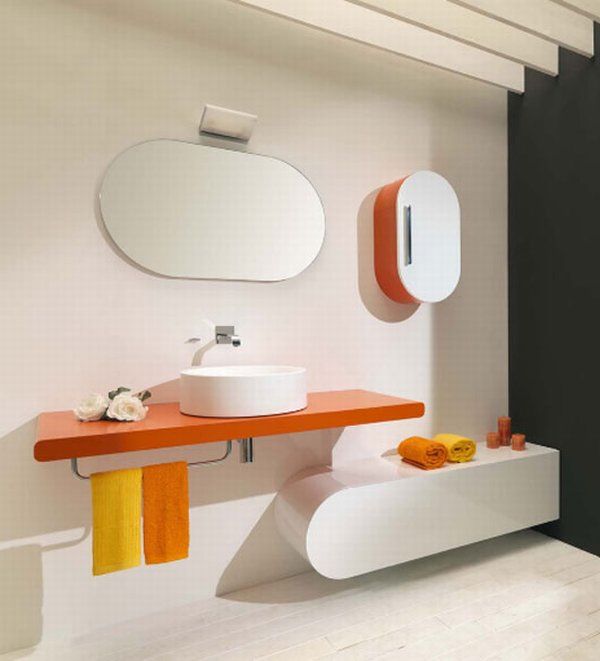This vibrant and modern bathroom features a sleek, white oval mirror centered on the wall, accompanied by an eye-catching, oval-shaped 3D light fixture just above it. The standout element is the bold orange countertop, which contrasts beautifully with the white basin sink and its contemporary silver faucet. To the left of the basin, a neatly folded yellow towel adds a pop of color, while an orange towel on the right complements the countertop. To the far right, a white seating area provides additional functionality, adorned with meticulously rolled orange and green towels for a refreshing touch. The setting is grounded by an adjacent black wall that adds depth and sophistication to the overall design.